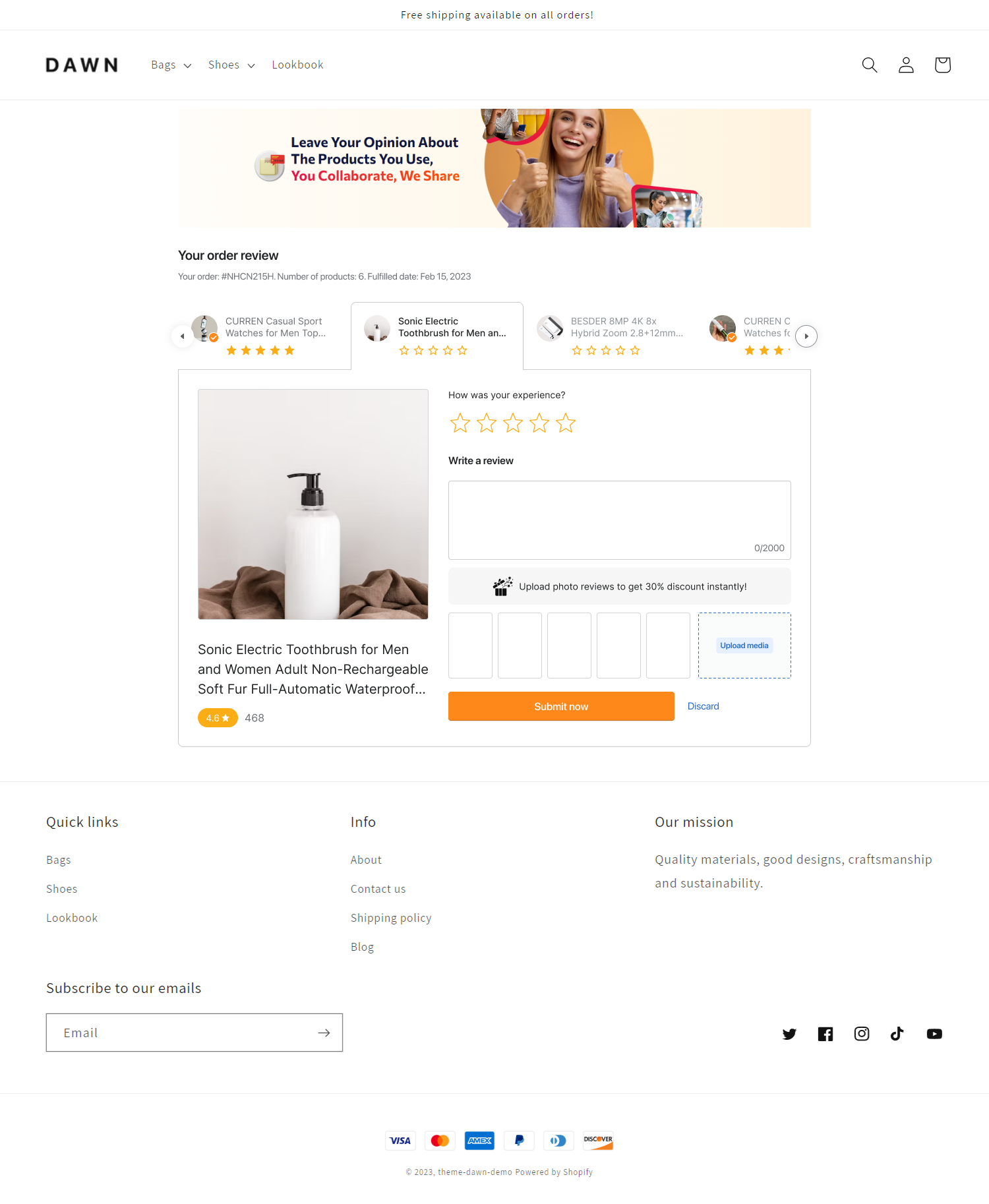The webpage for the online store "DAWN" features a sleek and modern design with a white background and black text. At the top, the DAWN logo is prominently displayed alongside navigation links for categories such as Bags, Shoes, and the Lookbook. Functional icons for search, account profile, and the shopping cart are neatly arranged at the top right corner.

Centrally located on the page, a bold announcement reads "FREE SHIPPING AVAILABLE ON ALL ORDERS." Just below, an engaging image of a smiling blonde woman giving two thumbs up visually represents customer satisfaction. Accompanying this image is a call-to-action message: "Leave your opinion about the products you use. You collaborate. We share."

Scrolling further reveals the "Your Order Review" section. Here, order details are displayed:
- Order number: NHCN2158
- Number of products: 6
- Fulfilled date: February 15, 2023

The products listed vary in rating, with some having a full 5-star rating while others are still open for review. Featured prominently is a "Sonic Electric Toothbrush for Men," which boasts a 4.6-star rating from 468 reviews. Customers are encouraged to write a review in the provided text box and can also upload photo reviews to receive a 30% discount instantly. The "Submit Now" button is brightly colored in orange, drawing attention to the next action for the user.

At the bottom, the page offers quick links and informational sections such as "Our Mission," which emphasizes values like quality materials, good design, craftsmanship, and sustainability. Social media icons connect users to various platforms, and a comprehensive list of accepted payment methods ensures a seamless shopping experience.

The cohesive design is accented with pertinent images, all set against a minimalist white backdrop, facilitating a user-friendly and visually appealing interface.